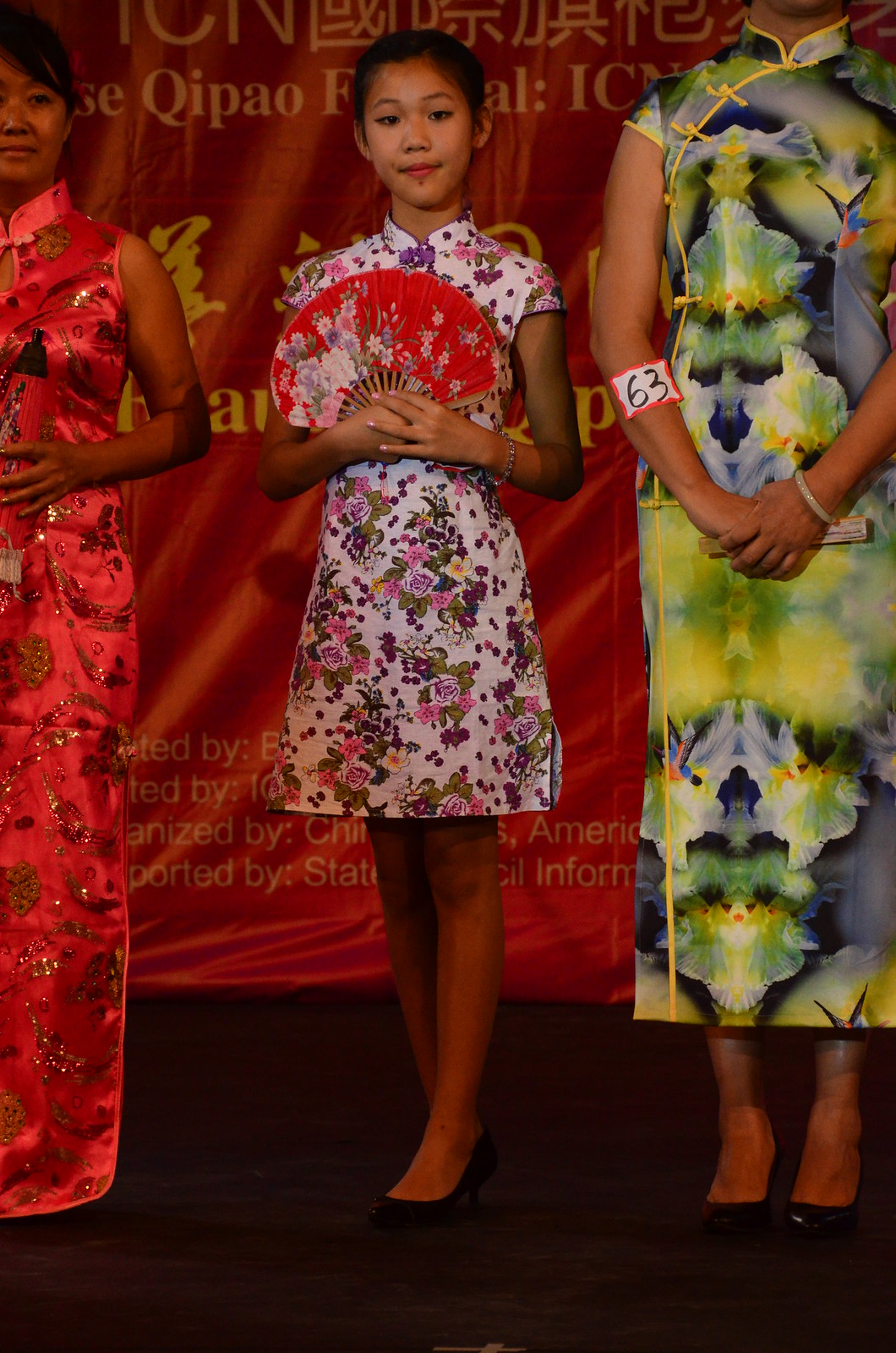The image features a young Chinese woman at the center, confidently smiling at the camera. She is adorned in a traditional white dress with short sleeves that reaches down to her knees. The dress boasts a vibrant floral print with hues of pink, purple, and yellow. Her black hair frames her face as she holds out a red hand fan intricately decorated with floral patterns. A bracelet delicately adorns her wrist. 

On her left stands a woman in a long, red, silk-like dress with gold decorations, whose black hair cascades as she gazes off to the right, holding an unidentified item in one of her hands. To the right of the central woman is another woman in a long, green patterned dress, marked with a white sticker bearing the number 63 in black text on her arm. 

Behind them stretches a red banner with yellow text, partially obscured by the central figure, adding to the festive atmosphere that suggests a traditional event or contest. The juxtaposition of traditional attire highlights the cultural richness and celebration of heritage embodied in the image.